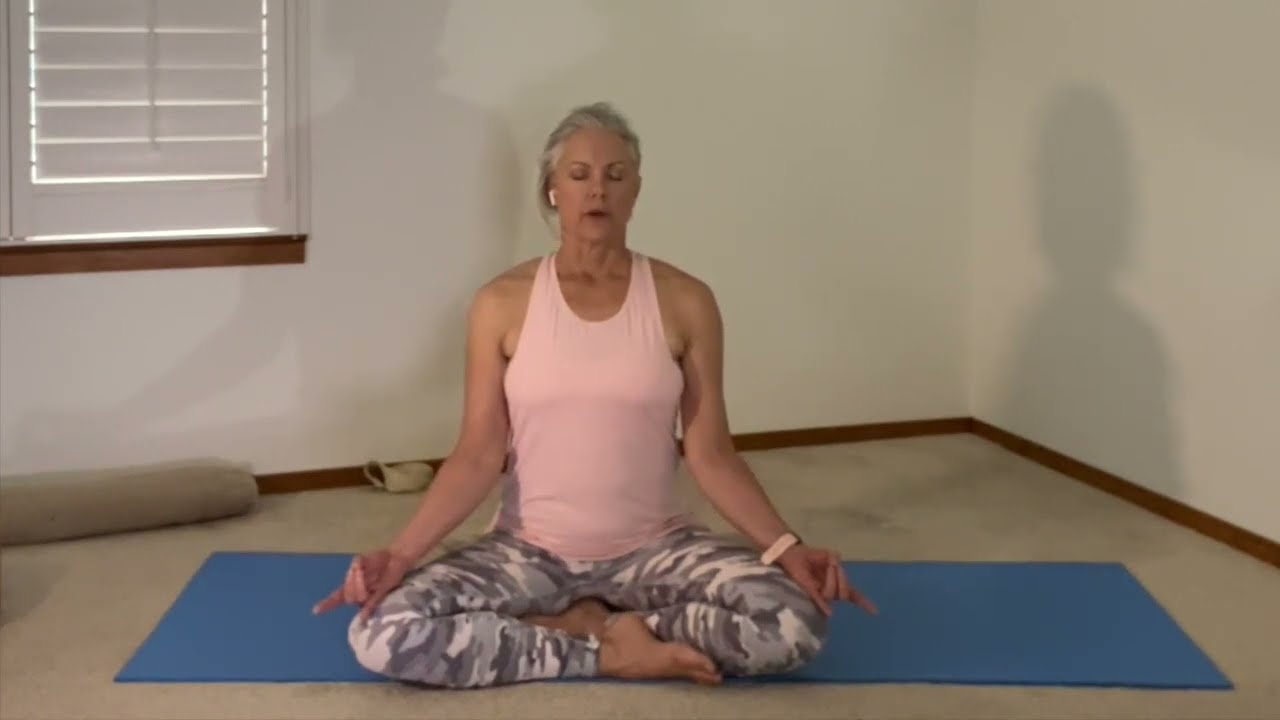In this photograph, an older woman is captured mid-yoga pose. The image, which appears to be a slightly blurry screenshot from a video, shows her seated on a blue rectangular yoga mat on a light beige floor. The setting is a simple room with white walls, a brown border along the bottom, and a shuttered white window with a brown windowsill on the left. She sits near the corner of the room, facing the camera with closed eyes and slightly open lips, as if speaking or chanting softly.

Dressed in gray camouflage leggings and a racerback light pink tank top, she has gray hair pulled back neatly. She sports a pink watch on her right wrist and a white earbud in her left ear, possibly following a guided yoga instruction. Her legs are crossed in a classic lotus position, with her knees pointing outward and feet drawn in towards the center. Her hands rest on her knees, forming a mudra with her ring finger and middle finger touching her thumb, while the other fingers extend outward. This serene moment is framed by the simple, uncluttered background, highlighting her focused meditation or yoga practice.